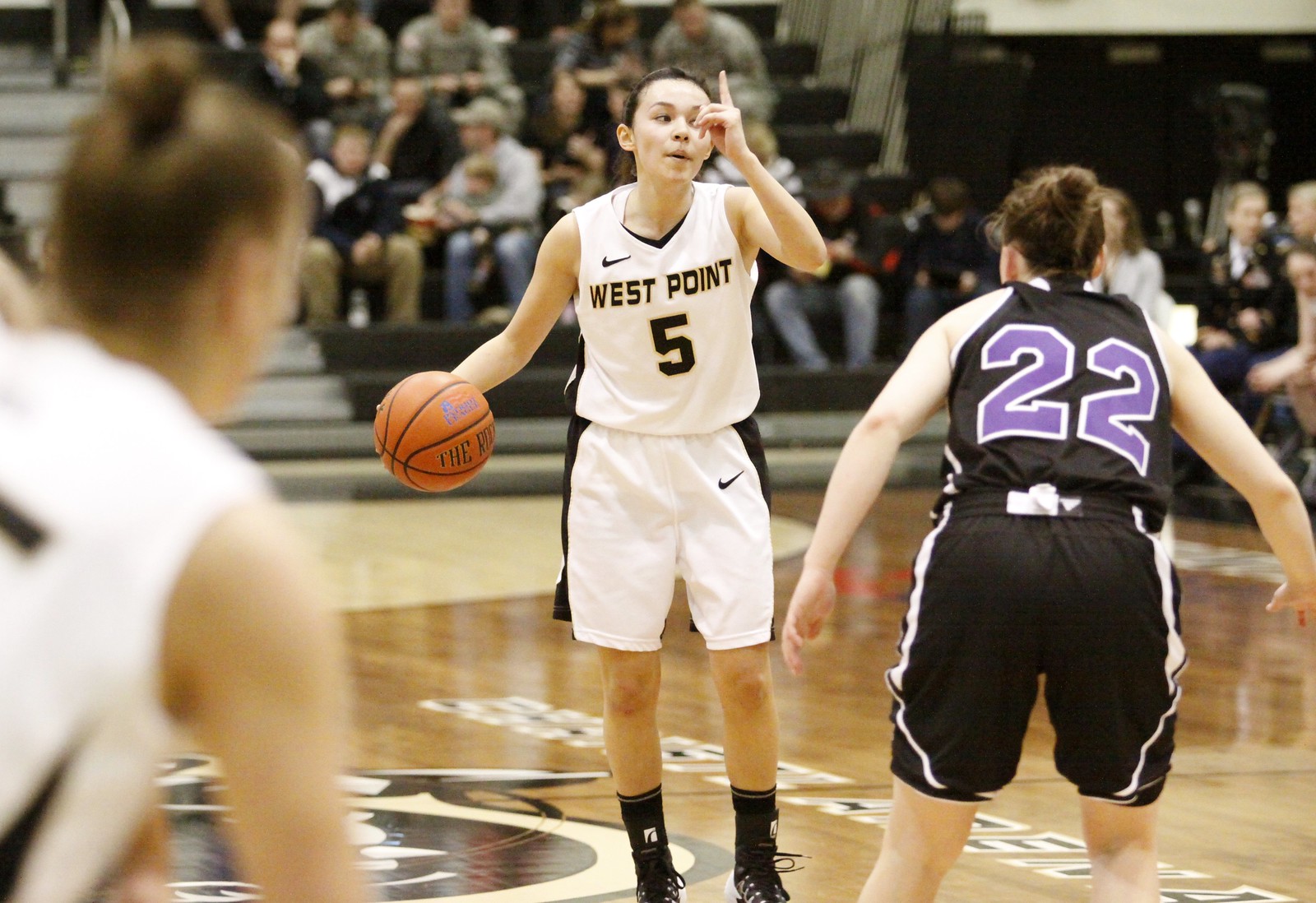The image depicts a high school girl's basketball game on a dark brown, shiny hardwood court. At the center of the image stands a player in a white jersey with black trim, emblazoned with "West Point" and the number 5, a black Nike swoosh visible on both the jersey and her white shorts. She has black socks and shoes, an orange basketball with black lines and blue and black lettering held in her right hand, while her left index finger points upwards, presumably signaling a play to her teammates. To the left, another player in white appears blurry and out of focus. On the right, a player in black with white trim wears the number 22 in purple on her back, crouched defensively, ready to guard or steal the ball. The background reveals several spectators seated in black bleachers, with a silver stairway to the left and more fans on the right, although the details are slightly blurry. A barely discernible logo adorns the center of the court.